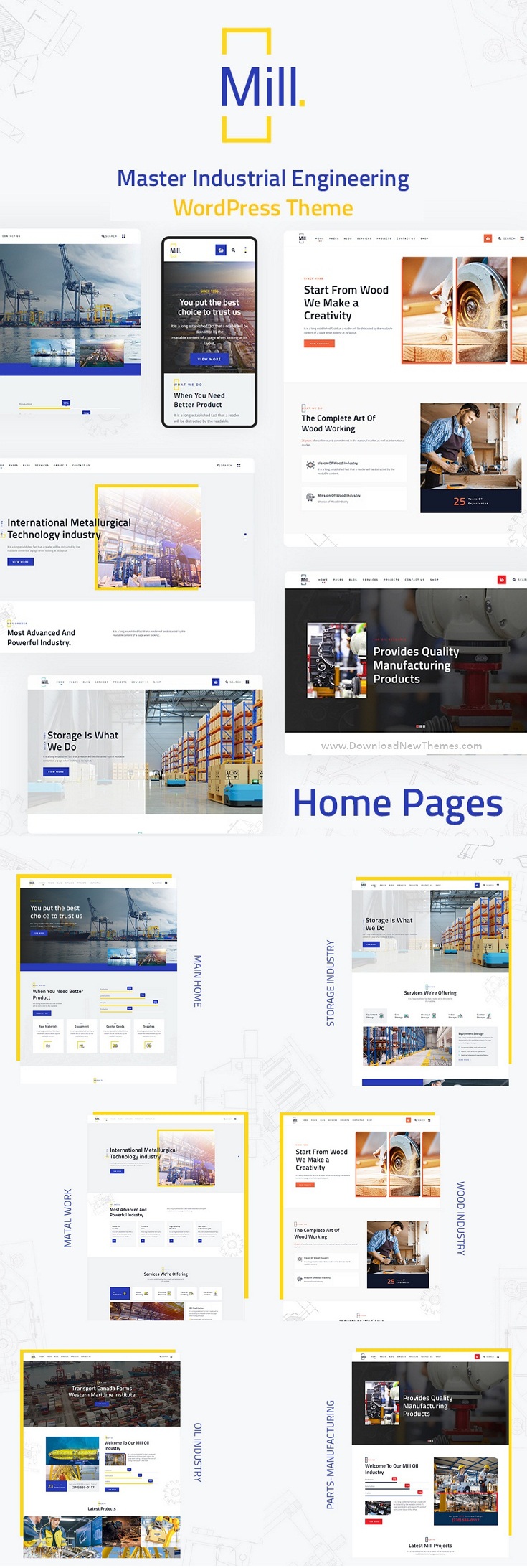The image showcases the emblem of the Master Industrial Engineering program, with the logo "M-I-L-L" prominently displayed in blue font. The acronym "AMI" is flanked by yellow square accents, both above and below, adding a distinctive touch to the design. Directly beneath the "Master Industrial Engineering" label, there is a reference to the "WordPress theme," indicating the context of the themes presented.

Below this header, the image features a structured layout, consisting of 11 distinct blocks arranged in a grid format. These blocks likely represent different WordPress themes, as suggested by the caption. The top block includes an illustration of a cellphone, while adjacent to it, there are blocks with a woodworking theme. Further along, several blocks depict warehouse environments. Notably, some of these themes are repeated, indicating their prominence or importance within the context of the image. Overall, the image combines elements of industrial engineering with digital theme representations, emphasizing a blend of tradition and modern technology.